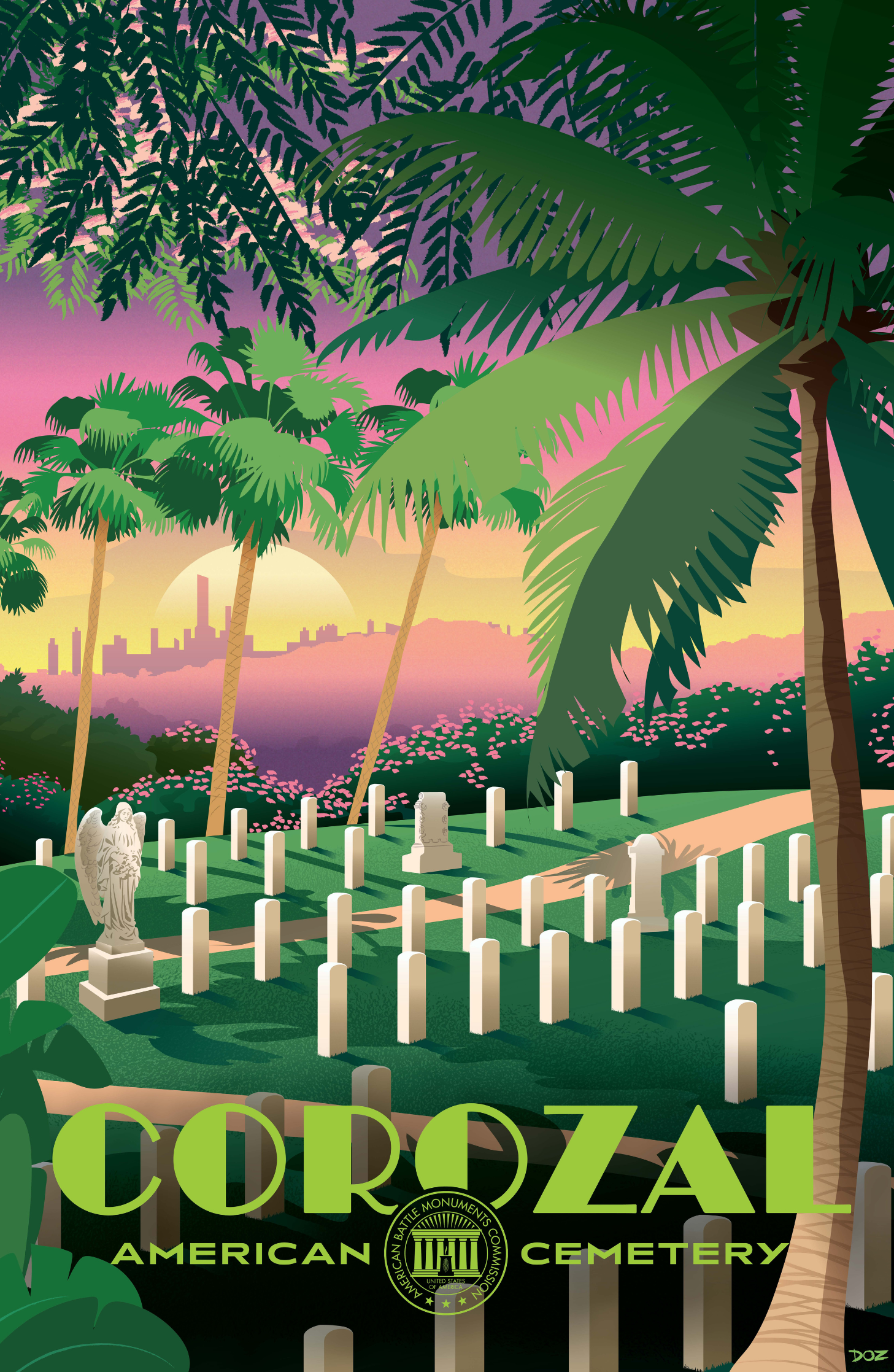This is a detailed and vibrant drawing of the Corozal American Cemetery, depicted with vivid colors and a blend of both simple and intricate elements. The foreground showcases deep green lawns dotted with a variety of vertical white headstones, some with unique shapes such as a square-topped and a cross-topped pedestal, and a prominent statue of an angel. Additionally, the cemetery features a well-defined brown walkway and clusters of pink flowers.

Palm trees, illustrated in 2-3 shades of green and brown, are scattered throughout the image, adding to the lush, tropical ambiance. The background is dominated by a city skyline under a strikingly colorful sunset. The sky features a vaporwave gradient transitioning from yellow near the horizon to a purplish haze, with the large, yellow setting sun casting its rays across the scene.

Further enhancing the detailed panorama, the base of the image includes text in capital green letters that reads "Corozal American Cemetery," alongside a seal with an image of a Greek temple, although the surrounding text is not legible. This image captures a serene, yet vibrant atmosphere, blending natural beauty with solemn remembrance.